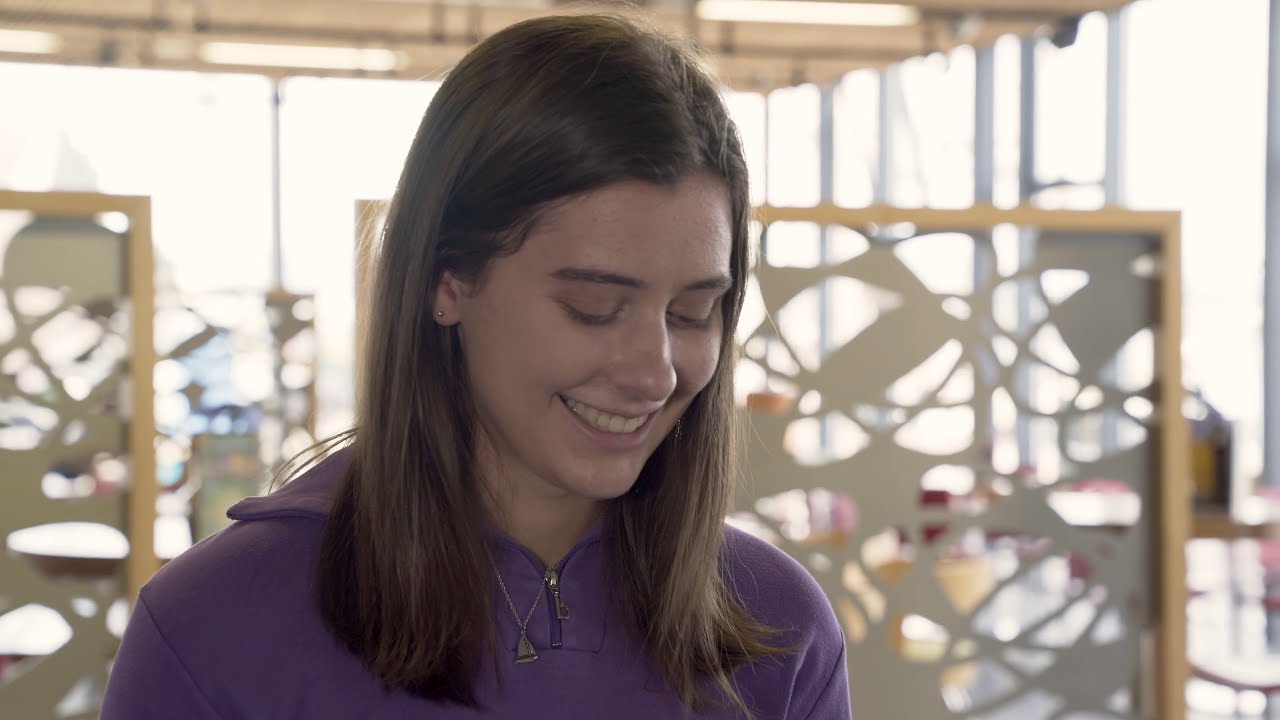The image features a young woman, likely in her late teens or early 20s, with straight brown hair that falls just past her shoulders and is parted on the side, tucked behind her ears. She has a warm, engaging smile showcasing her upper teeth, and her eyes are downcast, directed towards the ground. A small gold stud earring is visible in her right ear, and she wears a delicate silver necklace with a triangular pendant. She is dressed in a purple zip-up hoodie. The background, somewhat fuzzy and bathed in daylight, suggests an indoor setting, possibly a coffee shop or a restaurant. There are abstract cutout designs partitioning the area, framing abstract beige sculptures within wooden frames, all set against a mix of steel structures and a pinkish-white backdrop. She stands at the center of the photograph, looking down, evoking a serene and contemplative mood.